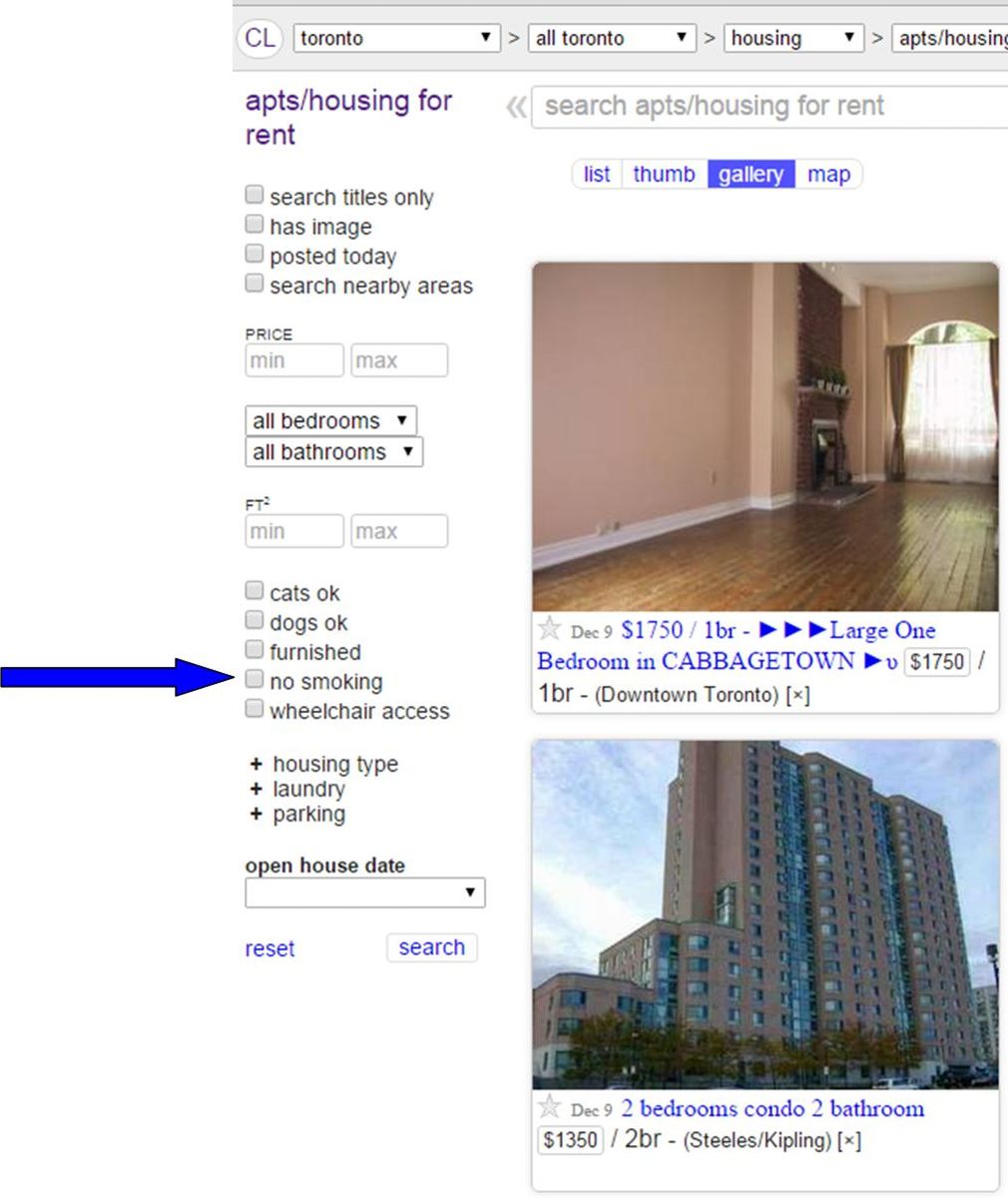This is a detailed screenshot from Craigslist showcasing housing listings in Toronto. At the top, there is a "CL" logo inside a white circle. The search parameters are set to "Toronto, All Toronto, Housing, Apartments / Housing." 

To the left side of the screenshot is a vertical menu with the following options: "Apartments / Housing for Rent," "Search Titles Only," "Has Image," "Posted Today," "Search Nearby Areas," "Price (Min, Max)," "All Bedrooms," "All Bathrooms," "FT (Min, Max)," "Cats OK," "Dogs OK," "Furnished," "No Smoking," "Wheelchair Access," "Housing Type," "Laundry," "Parking," "Open House Date," "Reset," and "Search." A blue arrow has been added, pointing rightward at "Wheelchair Access."

To the right, there are display options labeled "List," "Thumb," "Gallery," and "Map."

Below this menu, the first listing includes a photograph of a spacious, empty room. The walls are painted in a dusty pink hue, and there's a window at the back that allows sunlight to stream into the room. The details specify a one-bedroom apartment in Cabbagetown, available on December 9th, for $1,750 per month.

The second listing features a photograph of a tall apartment building. For this listing, the specifics mention a two-bedroom, two-bathroom condo located at Steeles / Kipling, available on December 9th, for $1,350 per month.